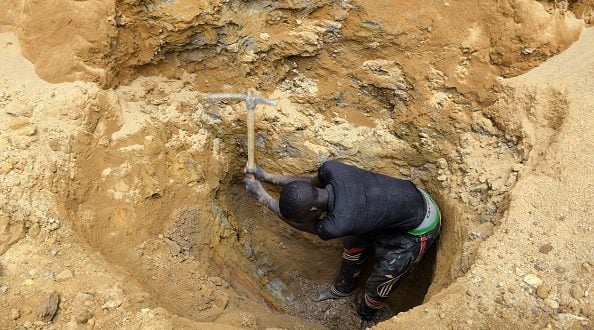In this image, a Black man is captured while holding a dark grayish pickaxe with a brown handle. He is dressed in a black shirt and black pants that feature a red stripe running down the sides and a green and gray waistband. Both of his hands grip the pickaxe firmly as he stands in a rounded ditch. The base of the ditch is composed of dark brown and darkish brown dirt mixed with grayish rock pieces. The ground near his feet is particularly rocky, with small brown and gray stones scattered around. The upper part of the ditch transitions into lighter, sandy brown soil, especially prominent towards the top right and left of the image.